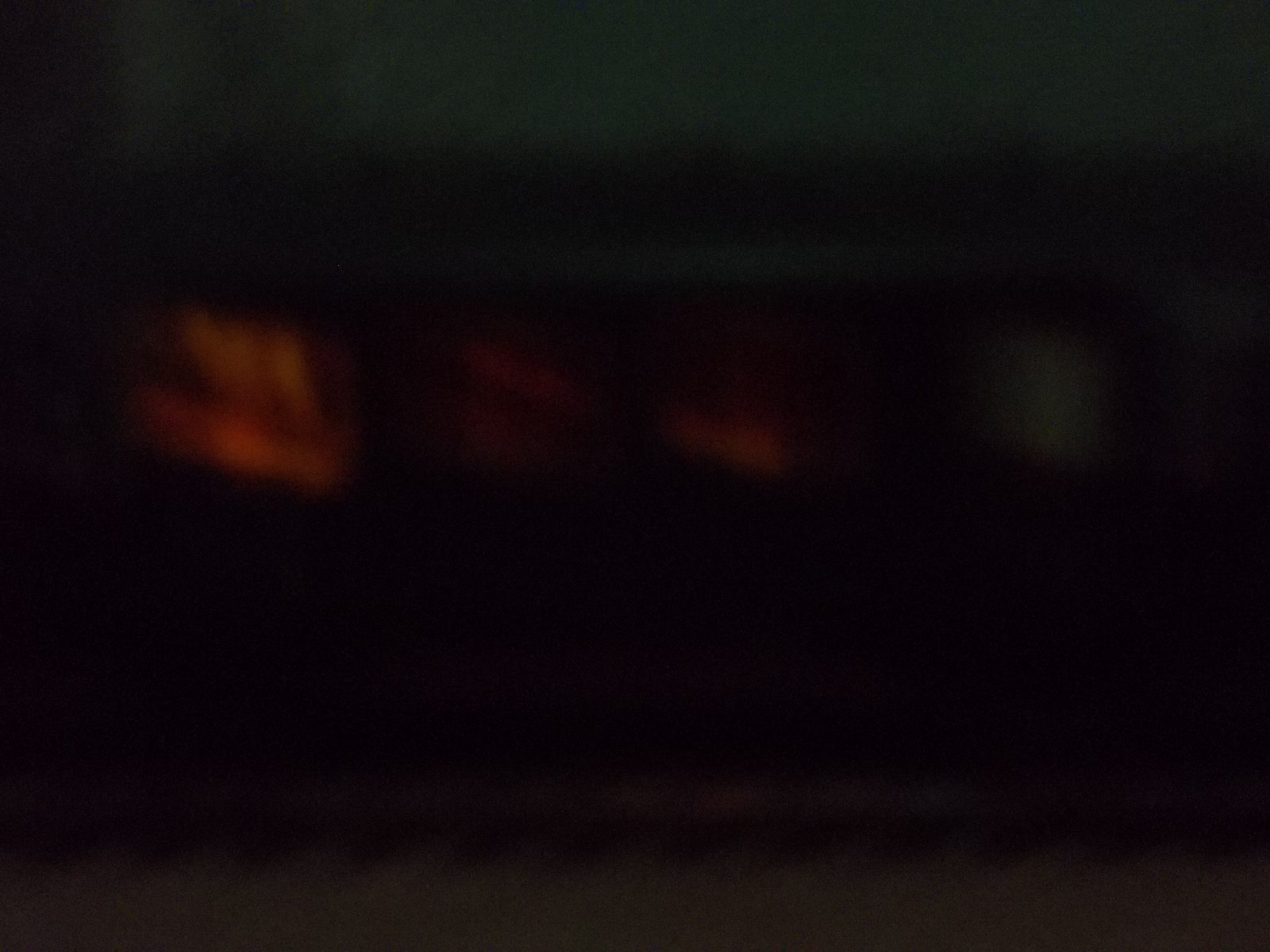The photograph is a very blurry, dark image that appears to have been taken at nighttime, making it challenging to discern specific details. The background is mostly a mixture of black and green, creating a shadowy ambiance. The focal point seems to be a large, rectangular object that predominantly appears black, although this could be due to the low lighting. There are red and orange spots visible on the object, possibly lights or reflections, adding to the ambiguity of the scene. Additionally, there is a white spot on the right side of the object. The image is grainy and indistinct, with any potential context or surroundings obscured by the darkness and low resolution.